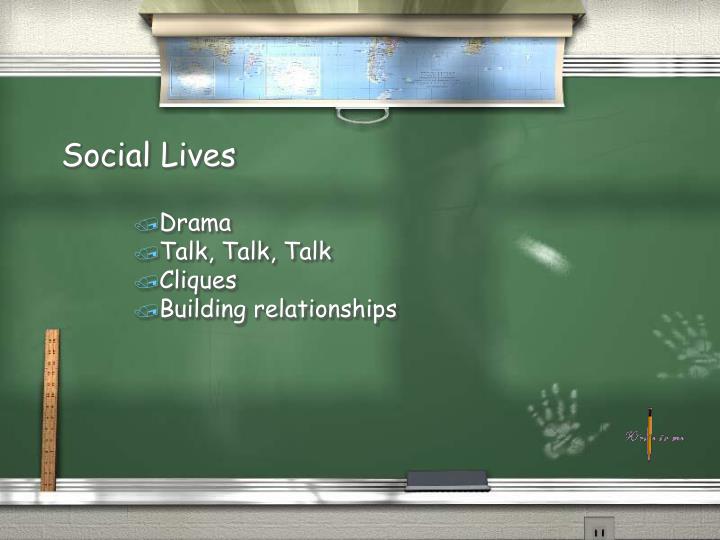The image appears to be digitally created and depicts a classroom scene dominated by a large green chalkboard, which takes up most of the visual space. Above the chalkboard, there's a partially pulled-down map with a light blue depiction of the ocean, framed by a white border and handle. Written on the chalkboard in white chalk are various lines of text: "social lives" at the top, followed by "drama," "talk talk talk," "clicks," and "building relationships," arranged vertically. On the bottom left of the chalkboard, a tan ruler stands upright, while on the bottom right, there are two white handprints. Directly below the chalkboard, there's a gray wall with a visible electrical plug. The colors present in the image include white, gray, blue, green, orange, red, brown, and silver, emphasizing a typical classroom setting.